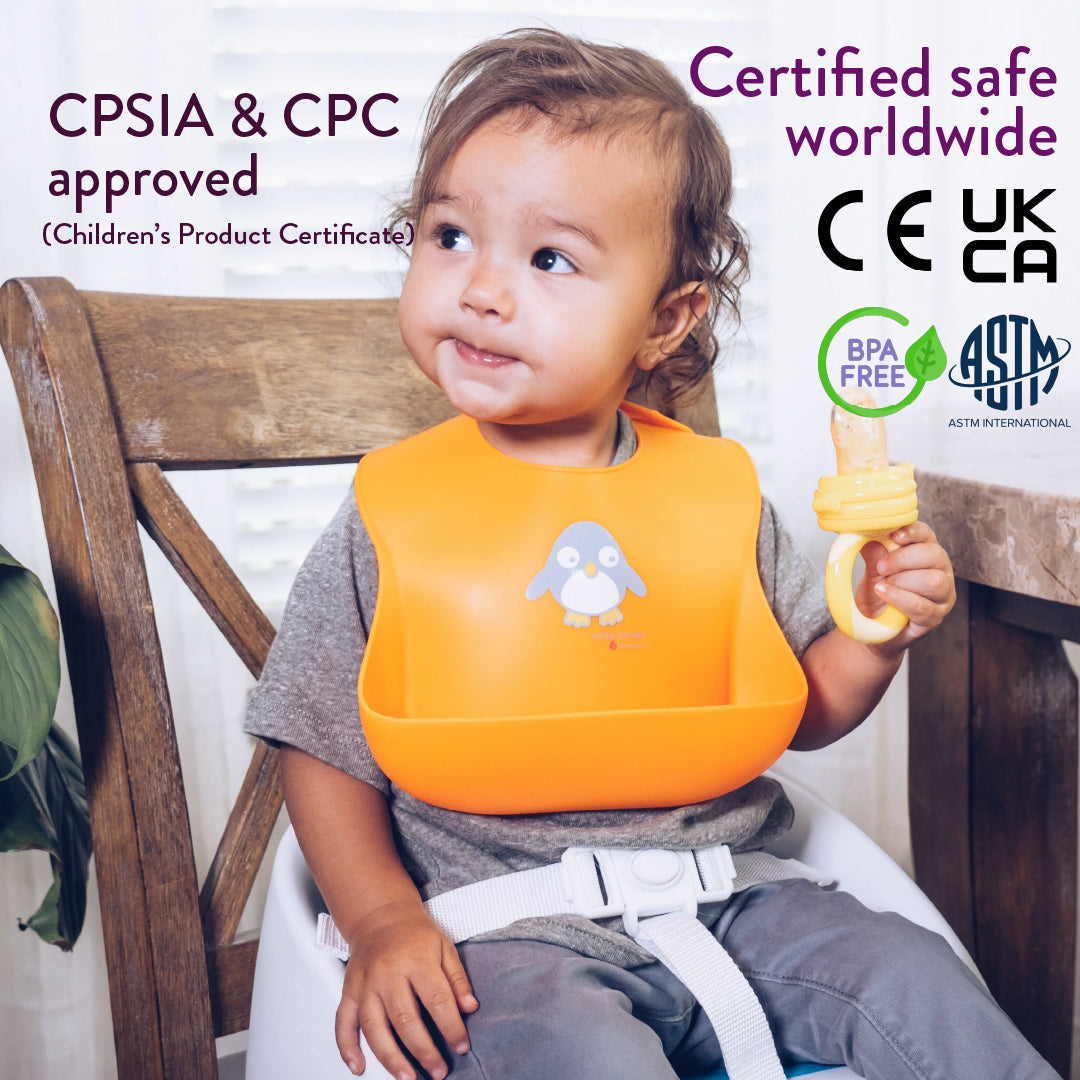This detailed image depicts an advertisement showcasing a young child seated in a white, securely buckled booster seat attached to a worn, wooden chair. The child, wearing gray pants and a gray short-sleeved shirt, is adorned with an orange, plastic bib featuring a penguin image and a crumb-catching pocket at the bottom. In the child's left hand, a yellow and white pacifier is held. 

The image is surrounded by various certification stickers and symbols indicating product safety. In the top left corner, the text reads "CPSIA & CPC Approved" with a note underneath specifying "Children’s Product Certificate." The top right corner displays "Certified Safe Worldwide" in purple letters, accompanied by the black text logos "CE," "UKCA," and "BPA Free" with a green vine encircling the BPA emblem. Additionally, "ASTM International" is prominently noted. 

The overall composition and detailed safety labels emphasize the product’s safety and certification credentials, ensuring parents of its compliance with numerous international standards.